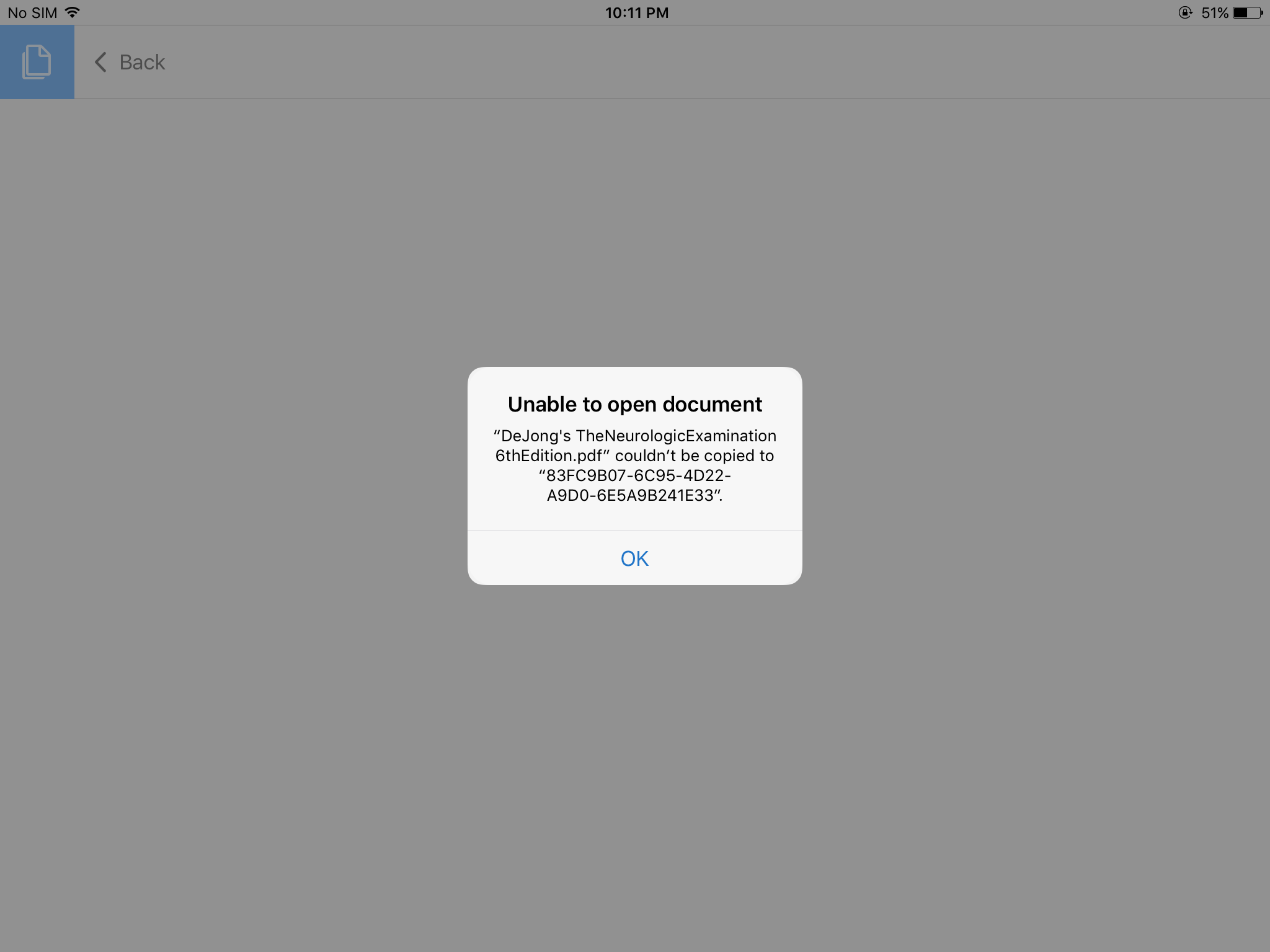A screenshot of an Apple device's user interface displaying an error message at 10:11 PM. The device, likely a tablet due to the absence of a SIM card, shows the battery status at the top of the screen. The error message states: "Unable to open document 'D Jones and Neurological Examination, 6th Edition.pdf'. The file could not be copied to a3fccc9b-07/c6c-5/4220/80a9d0/6e5a9b241e33." The message is highlighted in blue, and the background screen is dimmed, indicating that user action is required to proceed. The user must click 'OK' to dismiss the error and return to the main screen.